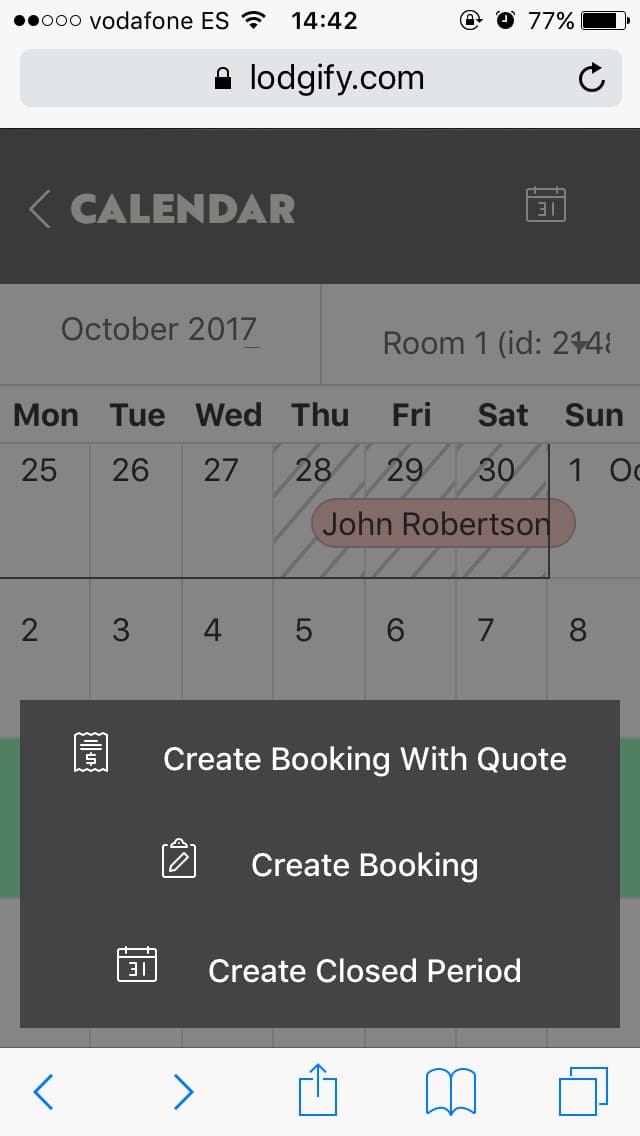The screen displays various indicators and information. Notably, the status bar shows "Tomplas" with two solid dots and three hollow ones, a Vodafone ES network signal, full WiFi connectivity, a clock displaying 14:42, rotation lock, and a battery at 77%. 

The screen includes a heading at the top that could possibly be related to "Logify.com" along with a refresh button and an unlock icon. Below, there's a calendar interface set for October 2017 showing "Room 1, ID," and the days of the week from Monday through Sunday. Dates visible include 25, 26, 27, 28, 29, 30, and 31.

A note specifies a task involving "John Robertson" with a number sequence "2345678." There's a gray section at the bottom indicating tickets, with an option to "Create Booking with Code." A clipboard icon signifies additional options beneath the "Create Booking" label, along with calendar controls for closing the period, a middle left arrow, right arrow, and an up arrow. There's also an open book icon and a series of squares representing various commands. The text mentions "20, 20, 30" several times and notes a shadowy filter effect on the interface.